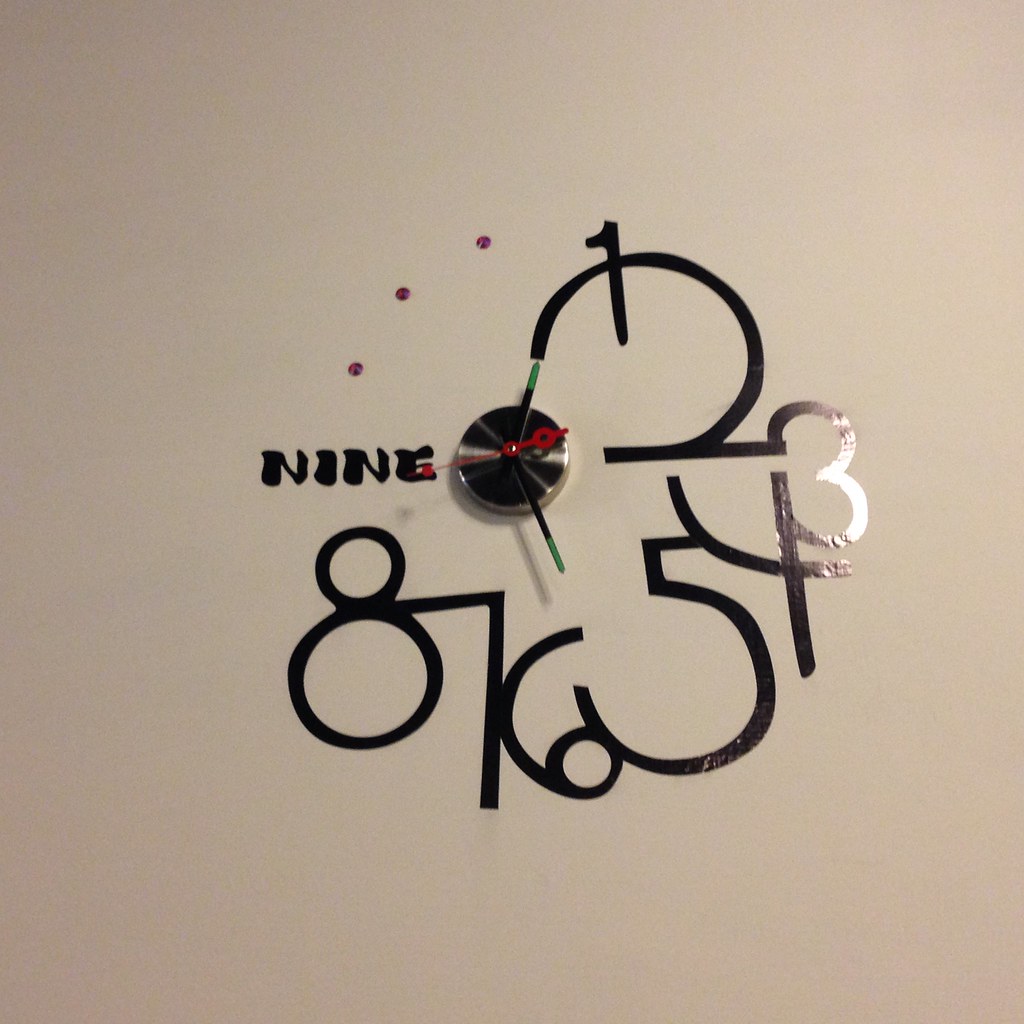This image depicts an abstract and artistic representation of a clock, creatively painted onto a wall. At the heart of the composition is a central mechanism featuring the clock's hands, which are the only mechanical elements affixed to the surface. The minute hand intriguingly points towards a series of unconventional markings that replace traditional numbers. These markings are artistically exaggerated and interwoven, defying conventional clock design. For instance, the numeral "2" is hyper-elongated and overlaps with the "1," while the "3" extends at a right angle from the central point, intersected by a "4" and accompanied by a "5." All these numbers are interconnected in a whimsical and unconventional style, except for the "9," which is uniquely spelled out in words. This clock serves as a piece of art rather than a functional timepiece, showcasing a blend of abstract creativity and visual intrigue.